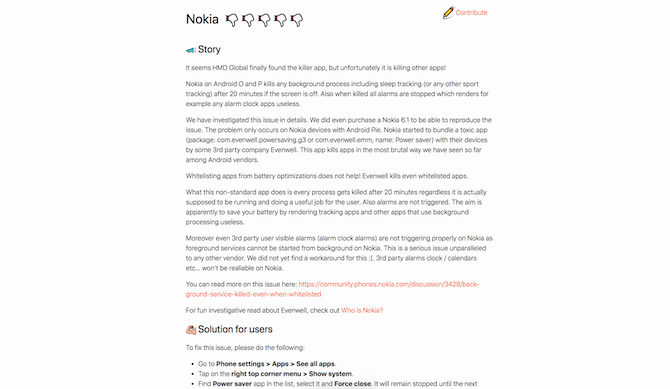On a white background in the upper right-hand corner, there is a red icon featuring the word "Contribute" accompanied by a pencil graphic. Below this, in black text, it reads "Nokia KNOKIA," followed by five thumbs-down icons. The central portion of the image appears blurry, but parts of the text can still be deciphered:

The story revolves around HMD Global seemingly discovering a "killer app," but unfortunately, this app terminates other significant background processes. Specifically, on Nokia devices running Android, all background applications, including sleep tracking apps, are halted after 20 minutes if the screen is off. This also disables alarms, rendering alarm clock apps ineffective.

Further investigation into this issue revealed that the problem exclusively affects Nokia devices with Android. Efforts included purchasing a Nokia 6.1 to replicate the problem. The issue is attributed to a bundled app with Nokia's Android devices, which aggressively kills apps and prevents background processes from functioning correctly.

Moreover, even third-party alarm clocks and calendar notifications fail reliably on Nokia devices because foreground services cannot be initiated from the background. This presents a serious and unprecedented issue among Android vendors, with no current solution for maintaining reliable alarm and calendar functions on Nokia devices.